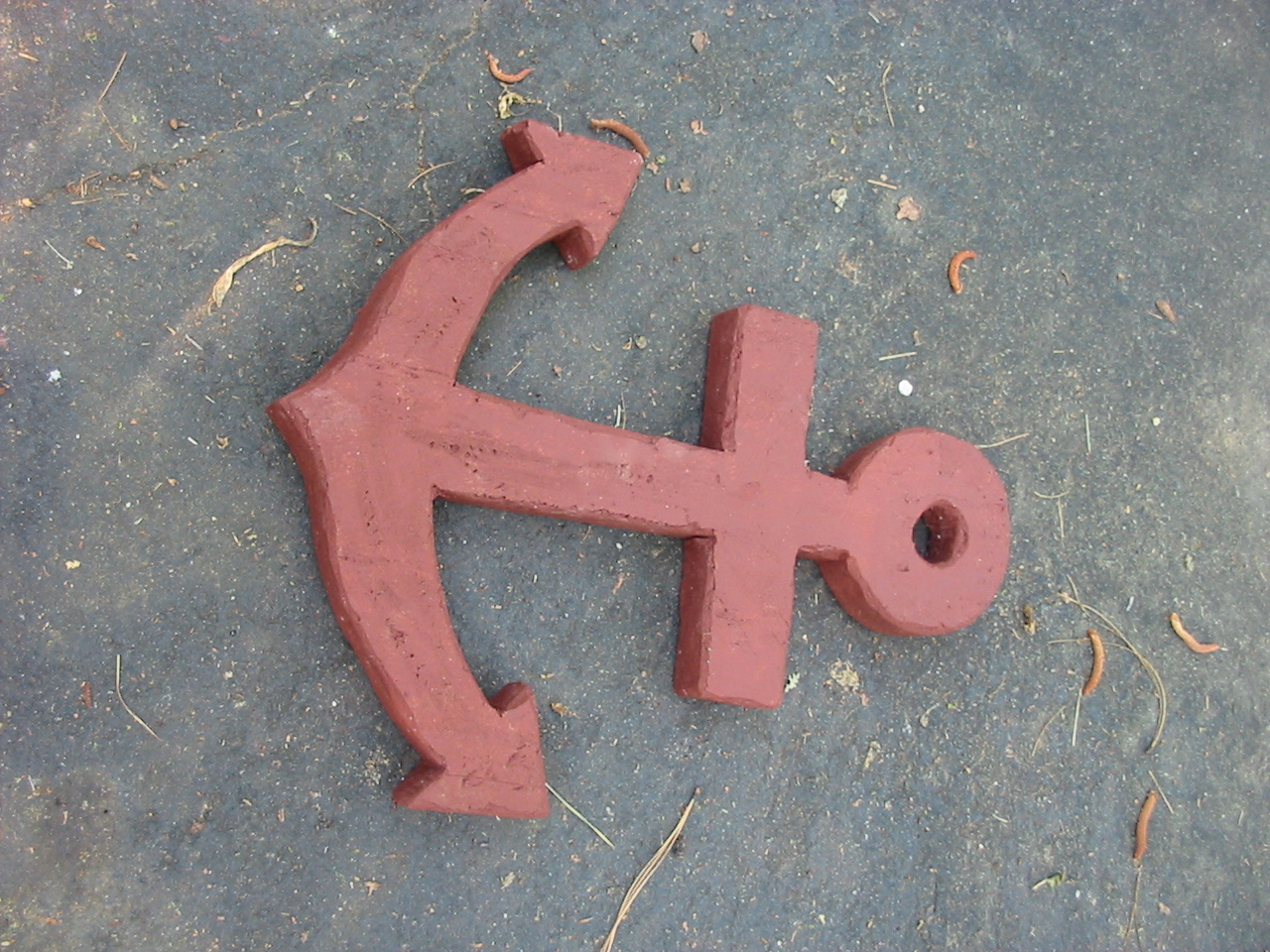This photograph captures a large, rust-colored red decorative anchor lying on a gray paved surface, possibly a driveway or sidewalk. The anchor, which appears to be made from wood, plaster, or a similar material, is positioned at a 45-degree angle to the left. Its base, shaped like an arrow, points leftward while the circular top with an eyelet designed for rope faces the right. The anchor features a cross-like structure with a bowed bottom and two upward-pointing prongs, adorned with arrow shapes. Scattered around it on the pavement are small plant debris, including twigs and grasses, indicating the outdoor setting and the influence of wind-blown materials. The photo's orientation and the sunlit environment add to the overall natural and rustic aesthetic of the scene.